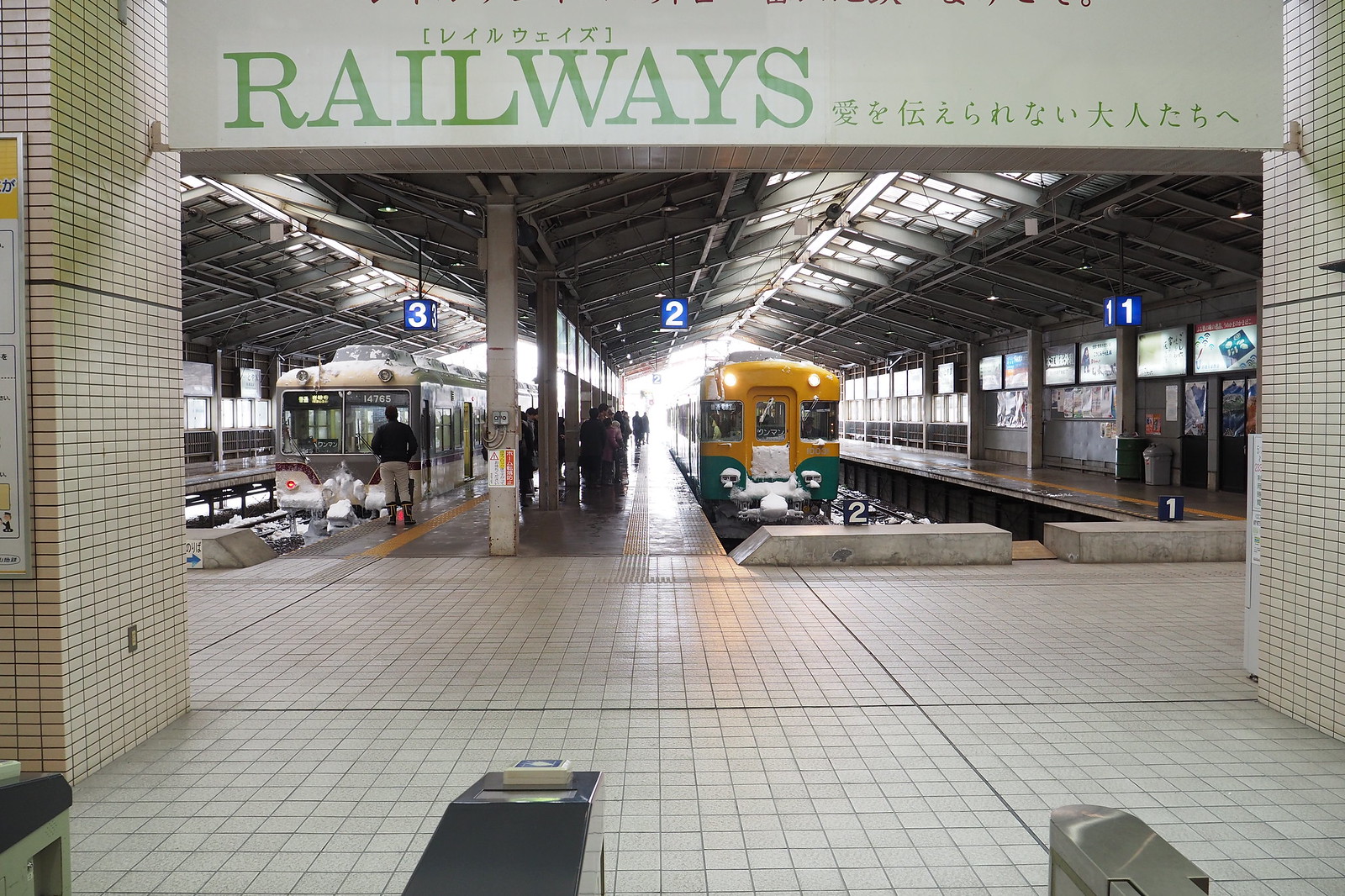In this detailed image of a train station, the focus centers on a vibrant, graffiti-style mural on the wall that reads "Railways" in green. Surrounding the English text are Chinese or Japanese characters, adding an international flair. The floor is covered in white, checkered tiles with distinct grout lines, and the areas are divided by blue, illuminated cube signs indicating platform numbers one, two, and three.

Currently, Platform 1 is empty, while Platform 2 hosts a yellow train with a greenish bottom, its headlights turned on. A group of people stands outside this train, awaiting entry. In the background, at Platform 3, another train with a beige top and a mixed stainless steel, maroon, and white bottom sits with a light dusting of snow covering its front.

Overhead, a metal roof shelters the scene, blending the indoor and outdoor aesthetics, while the ambiance suggests it could be an indoor-outdoor setup typical of many modern subway stations.